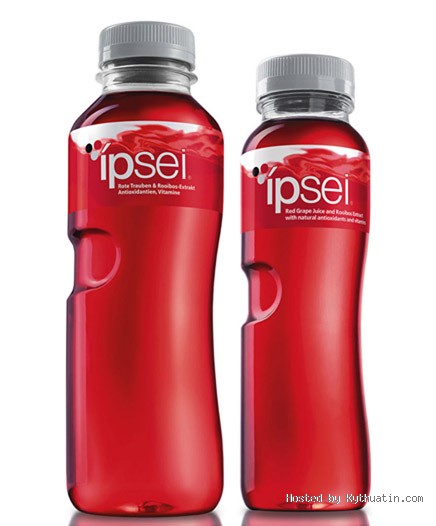The image features two bottles set against a plain white background. Both bottles share identical height, color, and label design. The bottle on the left is notably larger and wider than the bottle on the right. Each bottle is predominantly red with a gray cap. The label on both bottles reads "IPSEI." In the bottom right corner of the image, the text "hosted by kythuatin.com" is displayed in gray font.